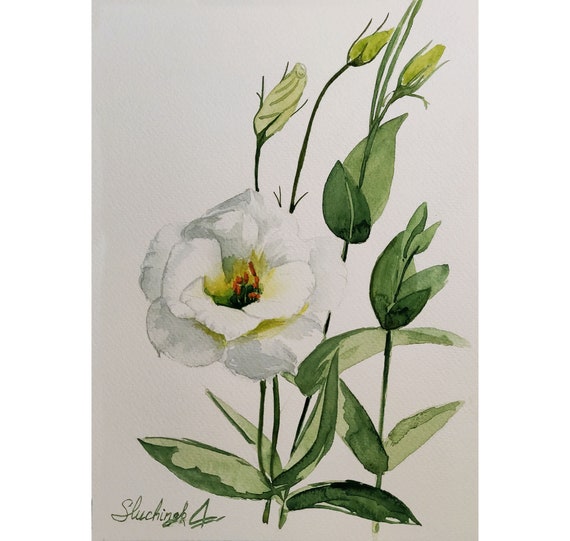The image is a delicate watercolor painting of a flowering plant against a soft gray background. The plant features three upward-reaching green stems adorned with leaves that exhibit subtle shading from light green to dark green. High on the stems are three buds yet to bloom, hinting at the cycle of growth. Below them sits a fully bloomed white flower positioned left of center, its seven petals elegantly framing a cluster of vibrant orange pollen pods. The flower's center hints at a soft transition towards yellow as it nears the core. Towards the bottom left of the painting, the artist's signature reads "Sleutchnik," accompanied by a prominent number four.